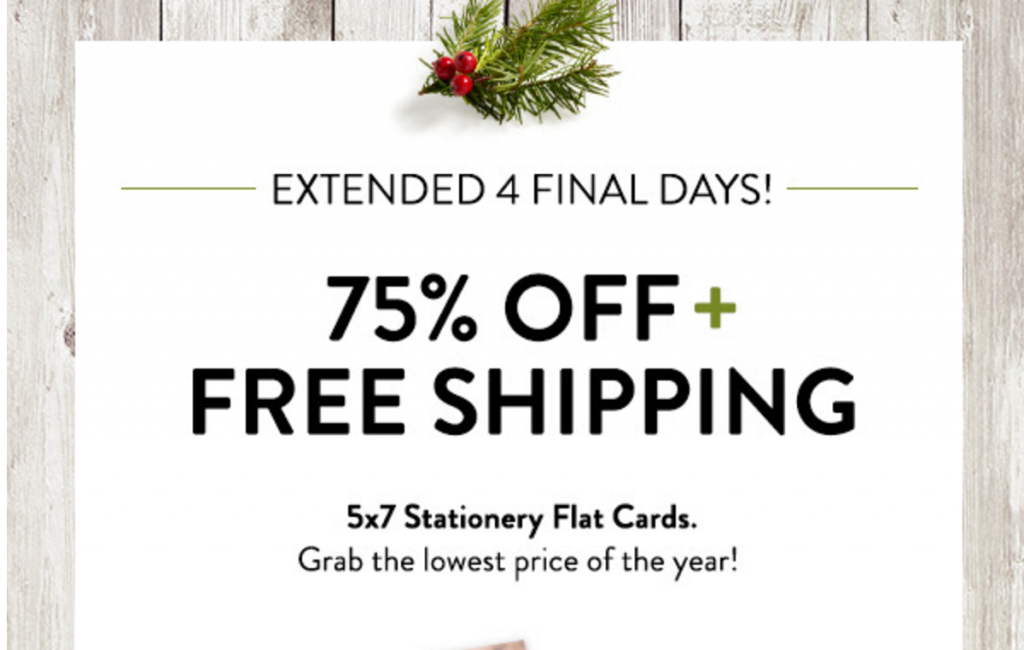The image features a background of gray wooden planks. Taking up most of the image is a large white rectangle, although it's cut off at the bottom, making its full shape unclear. At the top of the rectangle is an illustration resembling a green mistletoe with three red berries at its bottom. 

In the middle of the rectangle, bold black text announces, "Extended for Final Days" with "four more days" implied. This is flanked by a green line extending from both the left and right sides. Below this, more bold black text declares, "75% Off," followed by a green plus sign and the words "Free Shipping." Again in bold black text, albeit in a smaller font, are the details: "5 x 7 STATIONERY FLAT CARDS."

At the very bottom, bold black text urges readers, "Grab the lowest price of the year!" with emphasis added by an exclamation point.